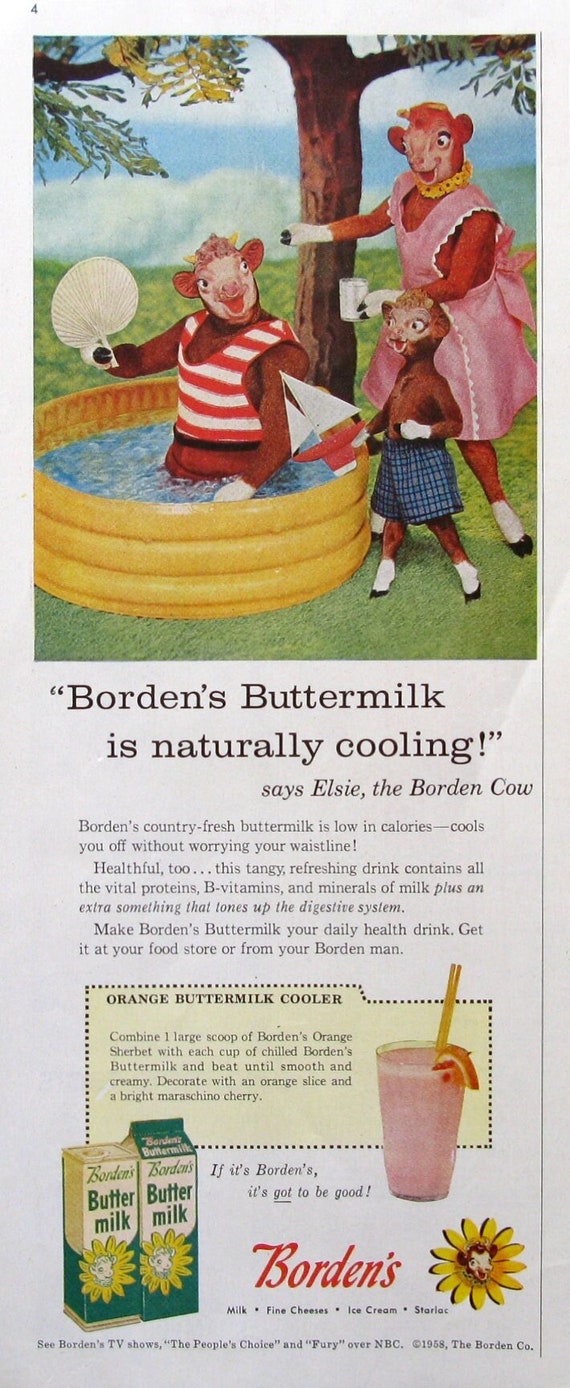This vintage advertisement for Borden's Buttermilk features a charming illustration of three anthropomorphic cows enjoying a sunny day outdoors. At the center of the scene is a male cow relaxing in a yellow kiddie pool, dressed in a red and white striped tank top and holding a white fan. Next to him stands a mother cow, elegantly attired in a pink dress and a floral choker, holding a glass of milk. A smaller, childlike cow wearing blue plaid swim trunks and clutching a sailboat stands beside her, gazing towards the mother and the pool. The backdrop includes a tree with green and yellow-tinted leaves under a clear blue sky. The ad headline prominently reads, "Borden's Buttermilk is naturally cooling," accompanied by an image of two cartons of buttermilk and a daisy logo at the bottom, identifying it as an offering from Elsie the Borden Cow.